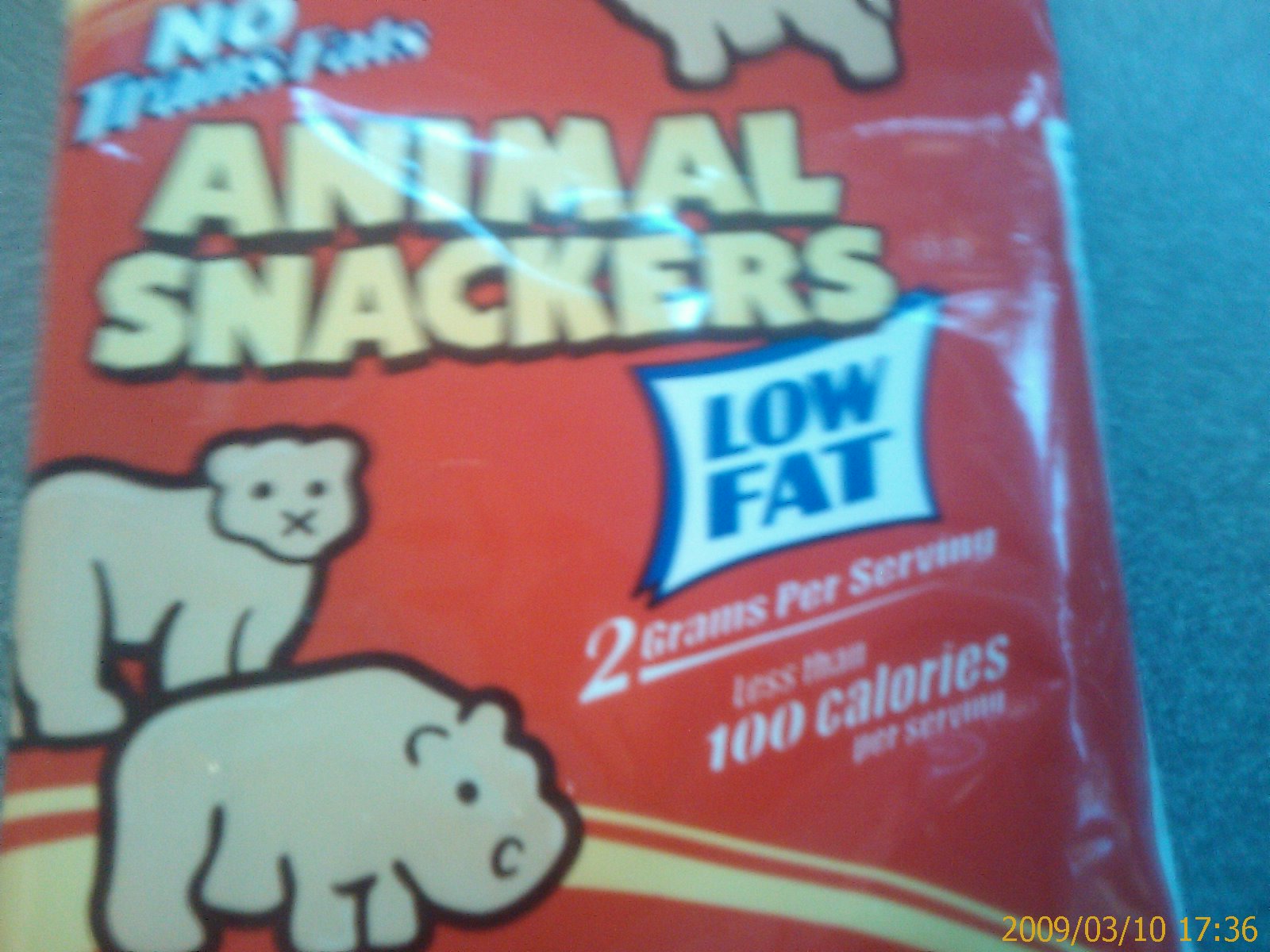This image, captured on March 10, 2009, at 5:36 PM (as indicated by the date stamp in the lower right corner), features a package of off-brand animal crackers titled "Animal Snackers." The background is a dark blue that contrasts with the vibrant red packaging of the snack. At the top left of the package, white text with a blue outline declares "No Trans Fats." The product name, "Animal Snackers," is prominently displayed in white with a black outline. Additional nutritional information states "Low Fat, 2 grams per serving, less than 100 calories per serving." On the left side of the package, illustrations of two animals, a gray tiger and a gray rhinoceros, are visible.